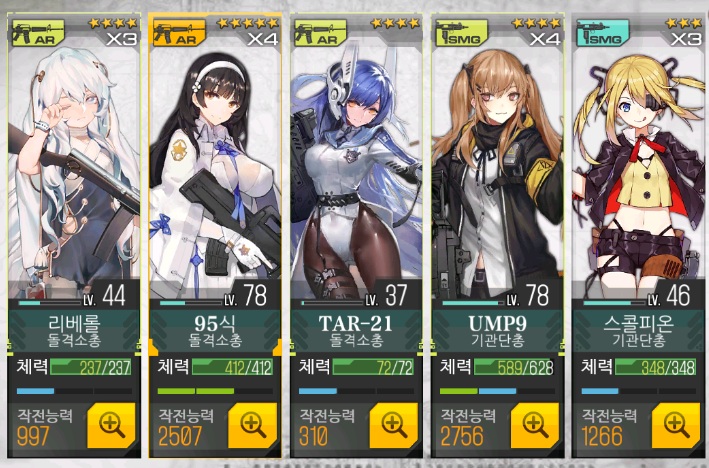This image depicts a mobile game interface showcasing the profiles of five female characters, each designed with an anime aesthetic. Each character card features detailed statistics, including levels, power numbers, and star ratings, set against a vertical layout that resembles collector or playing cards. From left to right, the characters are: 

1. A woman with long grayish-white hair dressed in a black dress, holding a rifle, labeled as AR (assault rifle) and rated 4 stars with a level of 44.
2. A dark-haired woman with a low-cut white top, a white robe, and a black rifle, also labeled AR, rated 5 stars with a level of 78.
3. A purple-haired woman in a white leotard, holding a weapon labeled AR, rated 4 stars with a level of 37.
4. A woman with black and yellow hair, wearing a black and yellow jacket over a white shirt, holding an SMG (submachine gun), rated 4 stars with a level of 78.
5. A blonde woman with pigtails, dressed in a black jacket over a yellow crop top and shorts, holding an SMG, rated 3 stars with a level of 46.

Each of the character cards displays various attributes, such as power rankings and specific weapon types, all marked with corresponding icons and numerical values. The characters' outfits are tight and somewhat provocative, with appearances suggesting they might be part of a squad with shared goals, possibly in combat or superhero capacities. The text on the cards appears to be in an Asian language, further emphasizing the anime influence.